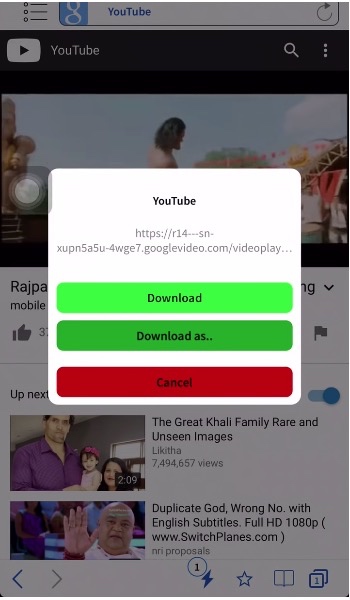In the center of this screenshot, captured from either a mobile or web application, there's a prominent white pop-up window displaying the black text "YouTube." Below this, a grey hyperlinked text is visible. The pop-up contains three buttons: a bright green "Download" button, a darker green "Download As" button, and a red "Cancel" button. 

The background scenery behind the pop-up resembles the YouTube interface, although it appears slightly different from the official YouTube website, suggesting that the site in question is accessing YouTube indirectly. A video is currently playing, and underneath, you can see a list of recommended videos queued next in the playlist. 

The overall design and functionality of this website seem geared towards downloading YouTube videos, giving off a somewhat dubious and potentially illegal feel.